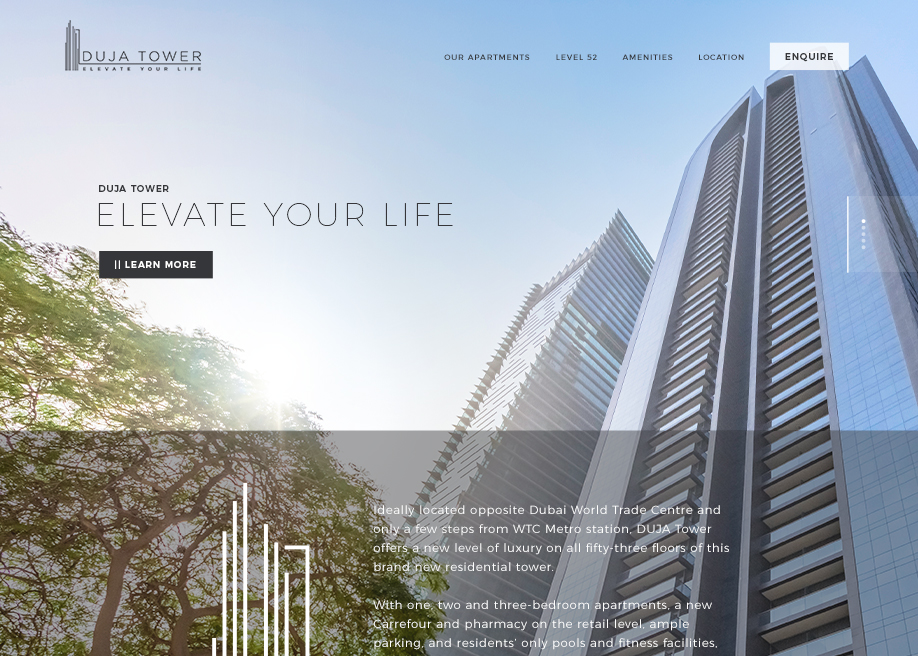This image showcases the homepage of an apartment complex website, featuring a visually striking background of two high-rise buildings captured from a low-angle perspective, giving a sense of their towering presence. To the left of the buildings, a substantial tree adds a touch of nature to the urban setting.

In the upper left corner of the homepage, the logo for "Doja Tower" is prominently displayed, accompanied by the slogan "Elevate Your Life." To the right of the logo, the navigation menu offers several clickable options including "Our Apartments," "Level 52," "Amenities," "Location," and "Inquire," providing users easy access to different sections of the site.

Central to the homepage, the text "Doja Tower, Elevate Your Life" is reiterated, accompanied by a "Learn More" button inviting visitors to delve deeper into the property’s details. 

Towards the bottom of the page, two informative paragraphs describe the property in greater detail. The text highlights the prime location of Doja Tower, situated directly opposite the Dubai World Trade Center and mere steps from the WTC Metro Station. The description emphasizes the luxury of the brand new 53-floor residential tower, offering one, two, and three-bedroom apartments, a care floor and pharmacy at the retail level, ample parking, and exclusive amenities such as residents-only pools and fitness facilities.